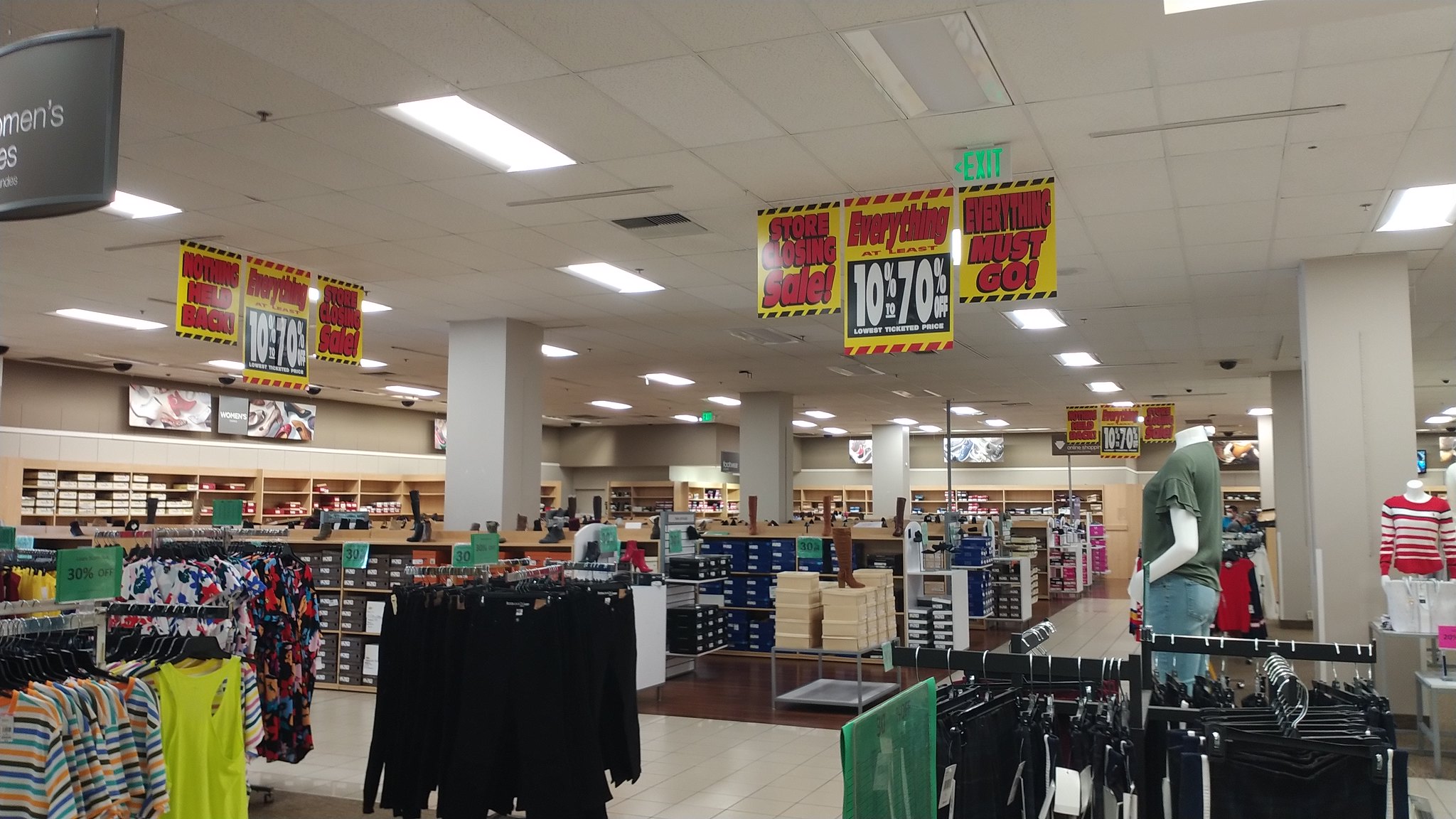This image depicts an angled view of a clothing section inside a department store, taken from the middle of an aisle. To the left, racks of clothing are visible, including striped short-sleeve shirts and a yellow tank top on a silver rack with multi-directional arms. Centrally, another silver rack holds pairs of black pants, while an adjacent black rack displays black pants with white stripes. Directly behind the black rack stands a headless mannequin wearing blue jeans and a short-sleeved gray shirt. Another headless mannequin, positioned on the far right and set atop a table, is dressed in a red and white striped sweater, with a white purse in front of it.

The store's white tile ceiling features flush fluorescent light panels and is adorned with several sale signs indicating a liquidation event; the central sign reads "everything 10-70% off," flanked by "store closing sale" and "everything must go" signs. These signs are repeated throughout the store, and an exit sign is seen hanging nearby. In the background, shoe boxes are stacked on wooden shelves lining the back walls and the center aisle. No shoppers are seen within the image, emphasizing the store's imminent closure.